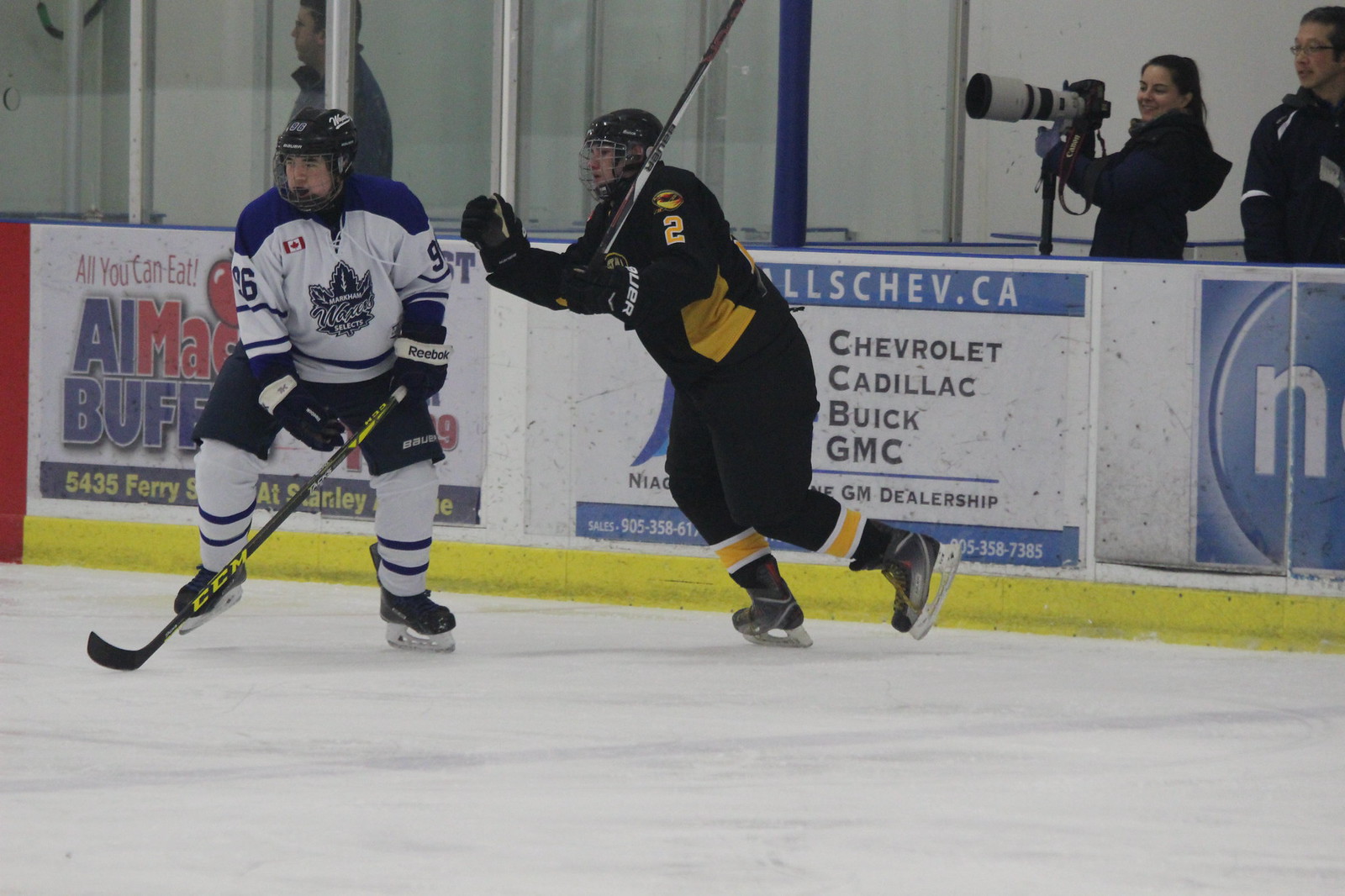This detailed photograph captures a dynamic moment in an ice hockey game, likely an amateur or semi-pro match given the absence of a large crowd. In the foreground, two players vie for control. Central to the shot is a player in a dark blue uniform with yellow stripes and the number 2, identifiable by his black helmet and black gloves. He is skating towards a nine o'clock position with his stick raised over his left shoulder and his right glove extended, seemingly poised to challenge or tackle his opponent.

To the left of the frame, another player faces us at a seven o'clock angle, possibly unaware of the approaching challenge. This player dons a white and navy blue uniform, with dark blue shoulder tops and white pants, and bears the number 96. His hockey stick is in contact with the ice.

The background includes advertisements along the wall—one partially promoting an "All You Can Eat" buffet and another referencing a GM car dealership. Just behind the glass, a photographer, dressed in casual attire, is seen aiming a camera with a large telescopic lens toward the players. She is flanked by two men, one to her right, and another further off, not directly observing the game. The ice's characteristic translucent, white surface and surrounding yellow stripe complete the setting.